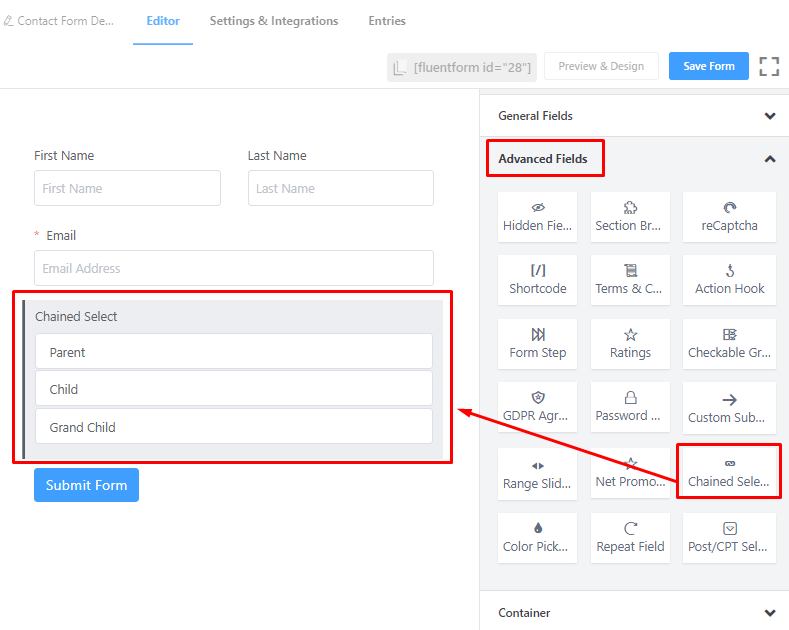The webpage displayed is a comprehensive contact form interface, showcasing several key sections arranged from left to right. The tabs include "Contact Form," "Edit," "Settings," "Integrations," and "Entries." Below these tabs is a highlighted border labeled "Fluent Form ID=28," indicating the current form in focus.

Next to it, there are options such as "Preview" and "Design," followed by a conspicuous blue button labeled "Save Form." Beneath these, users can input their personal information, including first and last names and email addresses. Highlighted in red is a "Chained Select" feature containing three dropdown entries: "Parent," "Child," and "Grandchild," which the user can fill out before submitting the form.

To the right, there's a dropdown menu labeled "General Fields," with another red-boxed section titled "Advanced Fields." This advanced dropdown has been expanded to reveal 18 tabs. One particular tab, also circled in red, is named "Chained Select." An arrow extends from this tab to the previously mentioned "Chained Select" box, clearly linking the two components within the form.